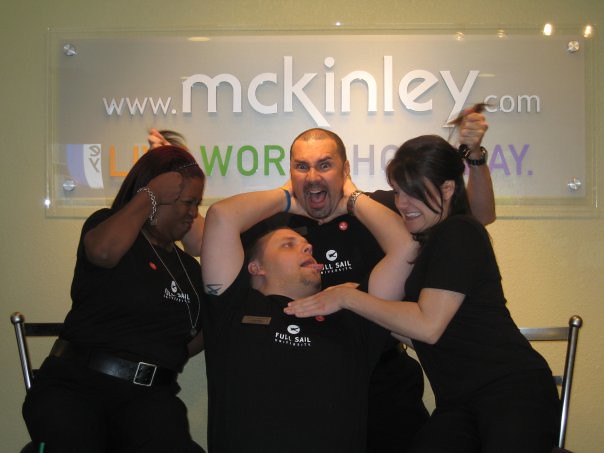The image features four people standing at the center, engaging in playful antics as they pose for a humorous photo. The individuals are dressed in black T-shirts that say "Full Sail University" and are miming various exaggerated actions like attacking and strangling each other, while all of them laugh and appear to be having fun. The setting seems to be indoors, likely a place of business, as suggested by a white wall in the background displaying a sign that reads "www.mckinley.com." Additional objects in the background include two silver chairs. The colors in the image include tan, gray, white, green, purple, orange, yellow, and silver. The overall atmosphere is casual and lighthearted, indicating a likely work environment where colleagues are enjoying a moment of camaraderie.